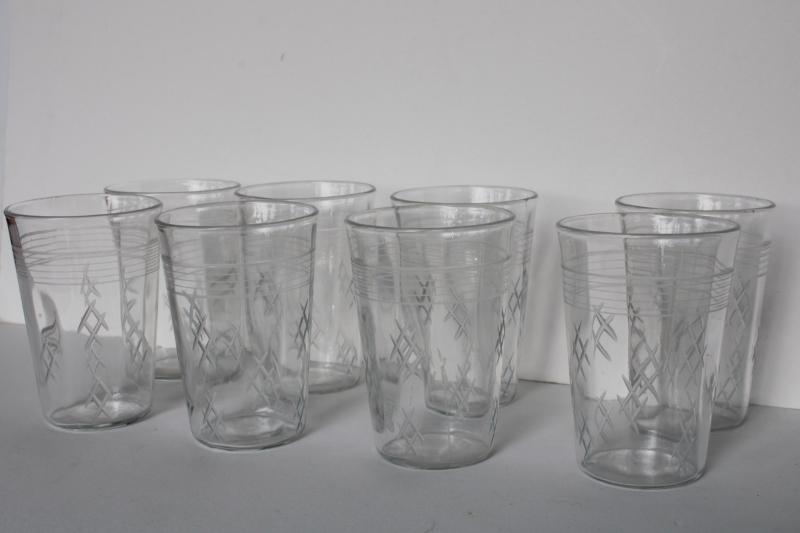The image displays eight identical, transparent drinking glasses arranged in two neat rows of four each. These glasses are placed on a slightly darker gray surface, against a gray wall, creating a monochromatic backdrop. The glasses feature intricate designs, consisting of intersecting lines that form hashtag-like patterns and rings near the lip of each glass. No contents are visible inside the glasses, and they sit spotless and clean, likely prepared for future use. A light source from the right side of the image casts subtle reflections on the glasses, emphasizing their clarity and precise arrangement.